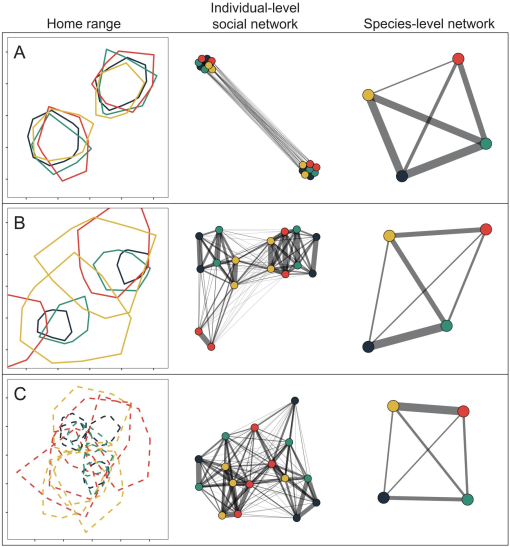This computer-drawn diagram, likely used in an educational setting or presentation, is organized into three main categories: Home Range, Individual Level Social Network, and Species Level Network. Each category consists of three vertically aligned sections labeled A, B, and C.

- In Category A:
  - The first block features various colored oblong shapes arranged in a square: red, blue, green, and yellow, in two sets.
  - The second block displays a straight line with small colored circles at each end.
  - The third block shows a square with an X in the middle, and different colors at each corner.

- In Category B:
  - The same oblong shapes from Category A are more spread out and connected with thin black cords.
  - An intricate pattern of squares with lines and small dots emanates from the central shapes.
  - The square with the X, now tilted, continues to show distinct colors in its corners.

- In Category C:
  - The shapes are represented in dotted lines.
  - A less chaotic but connected random pattern of the various shapes emerges.
  - The square with the X appears distorted, maintaining its colored corners.

Each block within the diagram offers a visual progression through the three described networks, underscoring the change in arrangement and connectivity of the shapes, dots, and lines from Home Range to Species Level Network.